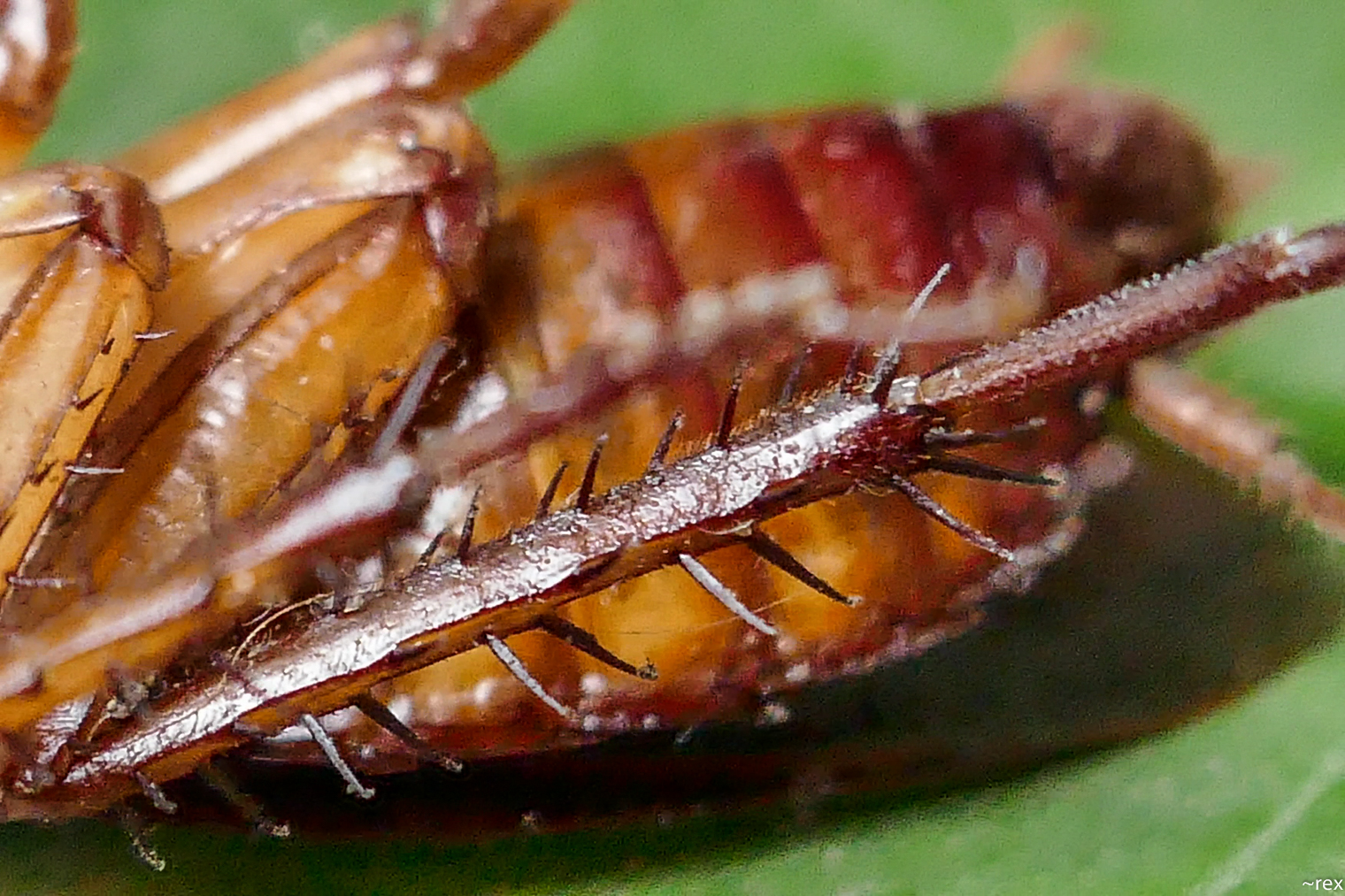A highly detailed, zoomed-in photograph captures the intricate features of an insect resting on a vibrant green leaf. The primary focus of the image is one leg of the insect, which dominates the foreground, stretching from the lower left to the upper right of the frame. This leg is dark, shiny, and adorned with small black spikes that run its length. The insect's body, seen in the blurred background, displays a variety of brownish hues, from tan to orangey-brown, with multiple ridges suggesting a shell-like structure and many layers. The insect appears to be overturned, with additional legs visible on the left side of the image. In the bottom right corner of the photograph, white text reads "teal day" followed by "R-E-X, Rex." The background is blurred, highlighting the green leaf's delicate veins where the insect is perched.